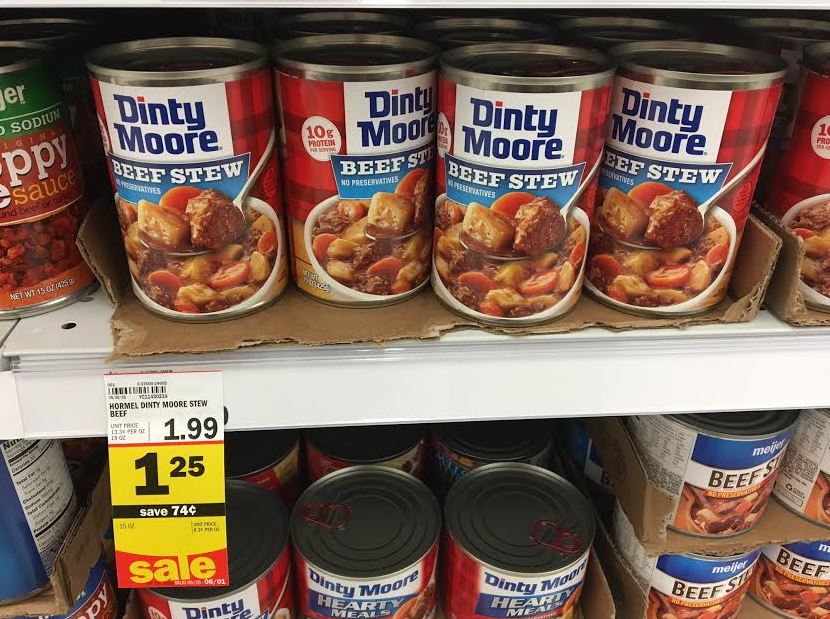This image captures an indoor scene of a grocery store aisle with two white shelves displaying various types of canned foods. The top shelf prominently features an open cardboard box base holding four neatly arranged cans of Dinty Moore beef stew. Each can, with a silver top, is wrapped with a distinctive red label bearing a white rectangle and 'Dinty Moore' in blue letters, except for a red dot over the 'i'. Adjacent to this, there's a white and red circle marking '10 grams protein' and a blue banner stating 'Beef Stew, No Preservatives'. Below the banner, a bowl of seasoned stew, complete with beef chunks, potatoes, and carrots, is depicted. A white tag attached to this shelf initially shows a price of $1.99 but is overlaid by a yellow sale tag indicating a discounted price of $1.25, saving 74 cents. The shelf below contains more Dinty Moore beef stew cans with the label 'Hearty Meals'. To the right of the Dinty Moore display, another brand with white labels featuring a blue rectangle that reads 'Meijer Beef Stew' is also visible.